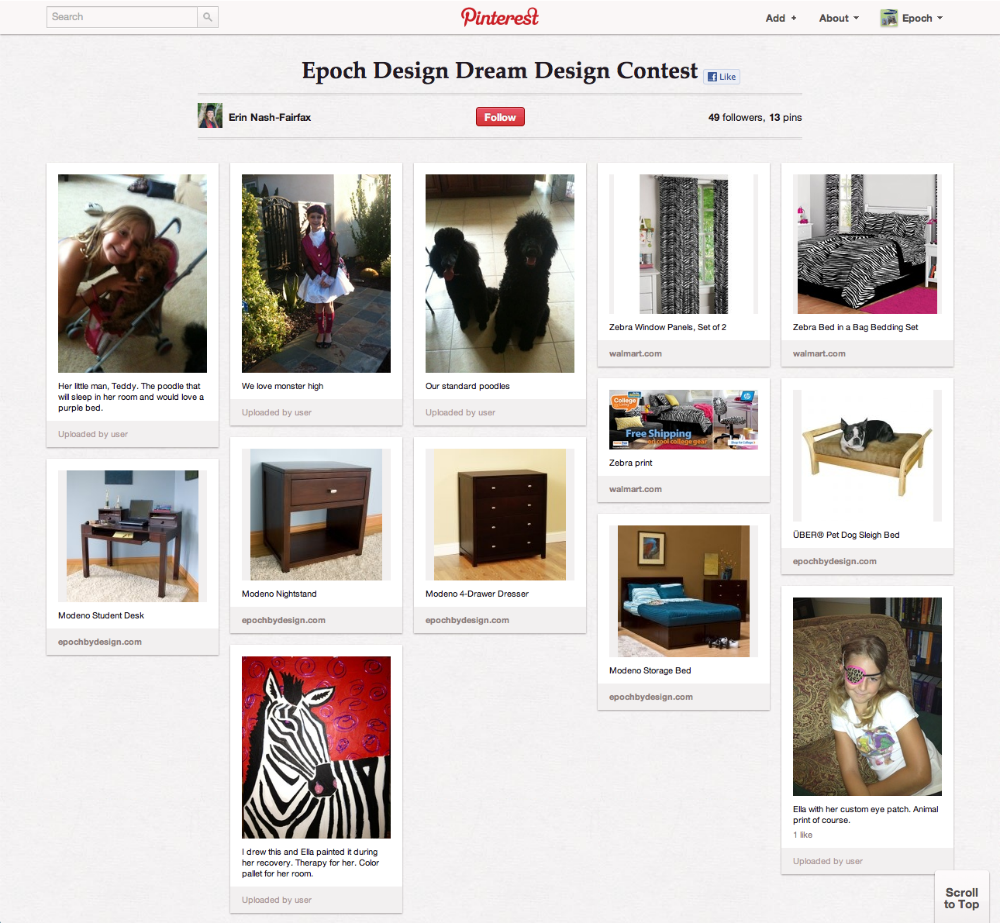The image shows a detailed webpage opened to Penris, featuring the Epic Design Dream Design Contest organized by Erin Nash Fairfax. Erin, identifiable by the red "follow" tab, has garnered 49 followers and has pinned 13 images showcasing her design ideas. Among the pins is a painted zebra, a collaborative artwork where Erin drew the outline and Ella painted it during her recovery therapy, reflecting the color palette chosen for her room.

Additionally, Erin has posted images of several Moderno furniture pieces, including a sleek desk, nightstand, four-drawer dresser, and a storage bed with drawers beneath the mattress. One picture highlights a little girl with her "little man" Teddy and her Poodle, who would adore having a purple bed. Their shared love for Monster High is noted, alongside their affection for their two large black Standard Poodles. The decor features a zebra-themed window panel set and matching bed-in-a-bag bedding set, and there is even an image of a miniature sleigh bed designed for a pet dog.